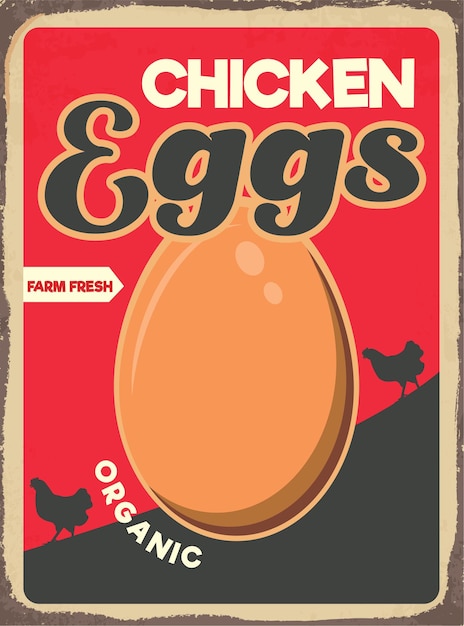This image portrays an eye-catching and colorful old-fashioned sign designed to look vintage. The sign, likely printed on metal and vertically rectangular, features a rustic and worn brown border with additional white framing inside it. The central background is primarily red, evoking a sky-like appearance, with black occupying the lower portion, reminiscent of the ground. 

At the top, in medium white font, the sign prominently displays the word "chicken," while below it, in larger bold black letters with a brown border, it reads "eggs." Centrally placed is a large, beige oval egg adorned with a white banner on its side, declaring “farm fresh.” Below the egg, the word “organic” is printed in bold white letters. Adding a whimsical touch are two black silhouette chickens positioned at the bottom edge, between the black ground and red sky sections, one on the left and one on the right.

Overall, the sign vividly advertises farm-fresh organic eggs, combining nostalgic charm with a clear and engaging layout.